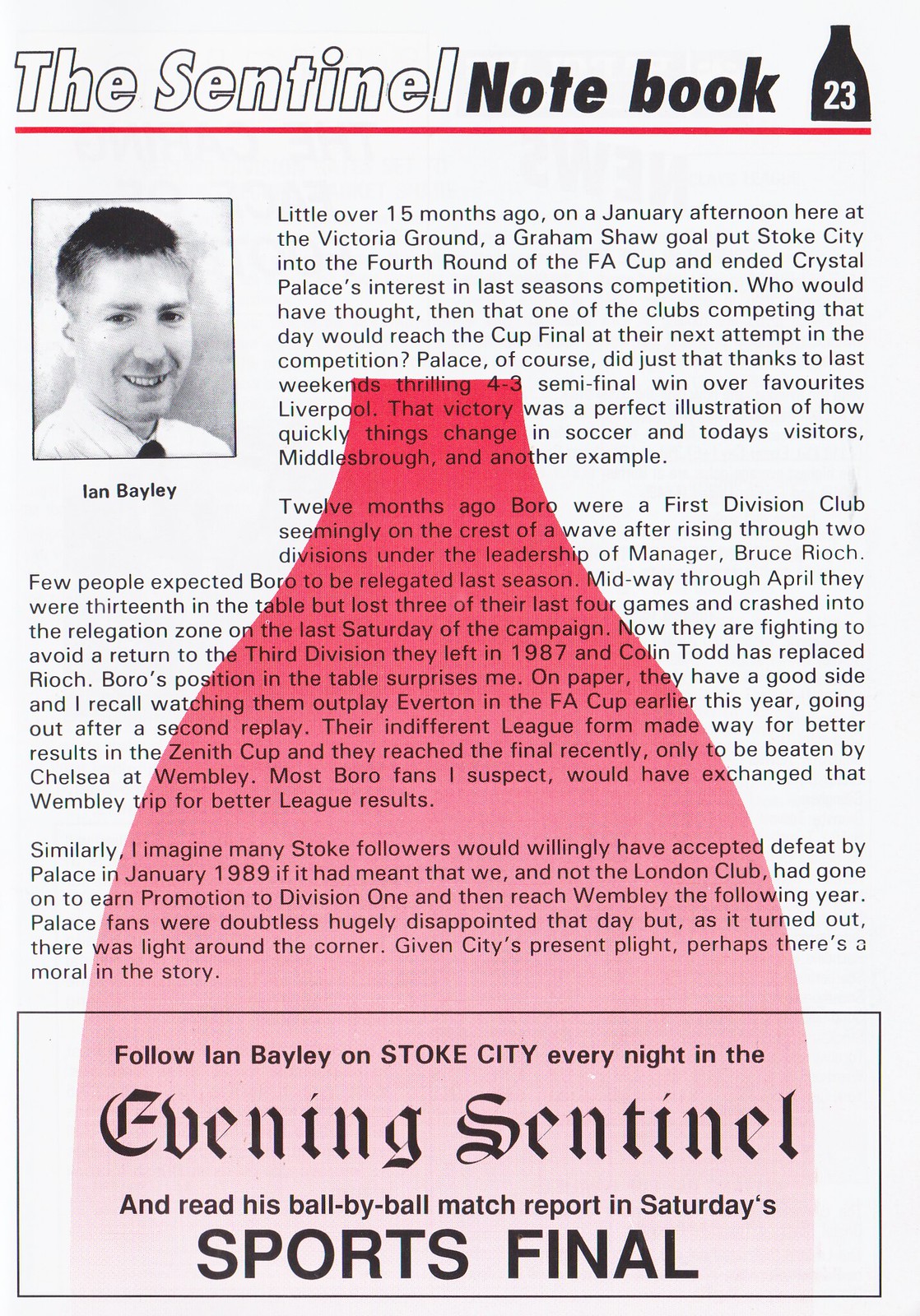The image is a page from a publication, likely a magazine or newspaper, titled "The Sentinel Notebook" and identified as being on page 23. It features an extensive article discussing notable soccer events. At the top left corner of the page, there is a portrait of Ian Bailey, a white man with short black hair, clean-shaven, wearing a white shirt, and a black tie. The magazine's name, "The Sentinel Notebook," is prominently displayed in contrasting white and black fonts, separated by a red line, and includes a distinctive logo resembling a bottle on the top, shown in black and watermark pink within the article.

The main article recounts events from over 15 months ago when a Graham Shaw goal at Victoria Ground advanced Stoke City to the fourth round of the FA Cup, ending Crystal Palace's chances. It highlights Crystal Palace's unexpected rise to the cup final in their next attempt, following a thrilling 4-3 victory over Liverpool. The narrative underscores the rapid changes in soccer fortunes, mentioning Middlesbrough's surprising relegation after a previously strong position and their subsequent struggles under new leadership.

At the bottom of the article, a boxed advertisement reads, "Ian Bailey on Stoke City every night in the Evening Sentinel," with the Evening Sentinel name in ornate black font, followed by a note to read his detailed match reports in Saturday's sports final, indicated in bold, large fonts.

The page is dominated by text, featuring colors like white, black, shades of gray, red, and pink, and has an overall style suggesting it is an excerpt from a larger book or magazine.